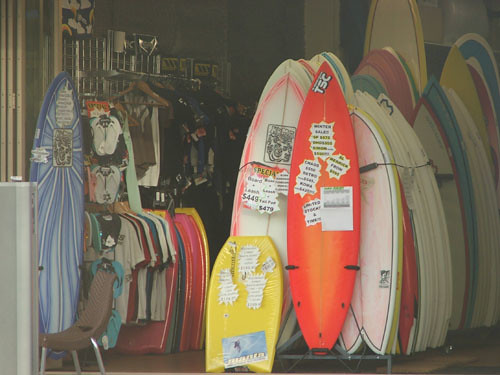This image depicts a surf shop, likely situated in a beachside community. Prominently featured are numerous surfboards of various sizes, shapes, and vibrant colors, stacked back-to-front, predominantly on the right side of the shop. Among these, a bright orange surfboard adorned with cartoon-like speech balloons and labels stands out. Additionally, an elaborate blue and white surfboard with intricate graphics is visible. Positioned towards the bottom center is a small, colorful boogie board. On the left side of the shop, racks of clothing are visible, including t-shirts and brightly printed vacation shirts, along with some sandals. Some t-shirts are white, red, and black, and the clothing items bear price tags. The setting appears to be dimly lit, giving the interior a somewhat dark ambiance. A small chair or stool can also be spotted amidst the merchandise.